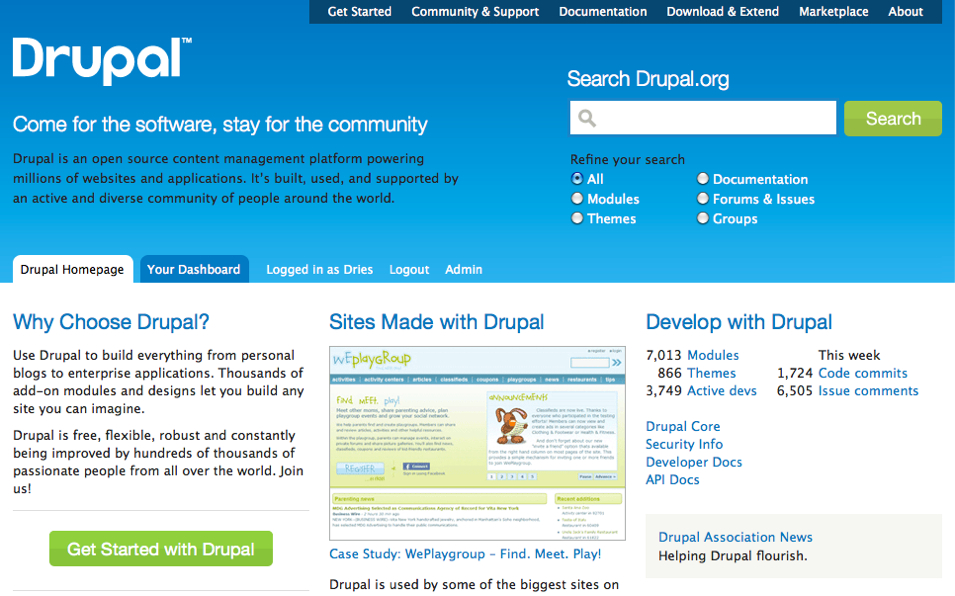**Website Screenshot Featuring Drupal Content Management Platform**

At the top of the screenshot, there is a blue banner displaying "DRUPAL™" in prominent white text, followed by a smaller tagline that reads, "Comfort, the software for the community." Beneath this, in smaller black text, it states: "DRUPAL is an open-source content management platform powering millions of websites and applications, built, used, and supported by an active and diverse community of people around the world."

Aligned from the center to the right of the top section, there are several main navigational menus labeled as follows: "Get Started," "Community and Support," "Documentation," "Download and Extend," "Marketplace," and "About," all in white text against the dark blue background. On the far right, a search bar is labeled "Search drupal.org" with a magnifying glass icon and a green "Search" button in white text. There's also a "Refine Your Search" option below, with buttons for filtering results by "All," "Module," "Themes," "Documentation," "Forums," and "Issues and Groups."

Further down, a section titled "Why choose DRUPAL?" in blue text explains the benefits of choosing Drupal for a variety of applications, from personal blogs to enterprise solutions. The accompanying text highlights Drupal's flexibility, robustness, and the passionate community contributing to its development. A prominent green button encourages users to "Get Started with DRUPAL."

In the center, the section "Sites Made with DRUPAL" provides examples and case studies, mentioning notable sites like "WePlay Group" and "FindMePlay." Additionally, on the right, a statistics panel showcases key Drupal metrics: 7,013 modules, 866 themes, 3,749 active developers, 1,724 code commits this week, and 6,505 issue statements. The section includes further navigation options such as "Procore," "CIrc Security Information," "Developer Docs," and "API Docs."

This cleaned and detailed caption gives a thorough overview of the visual elements and textual content presented in the screenshot of the Drupal website.